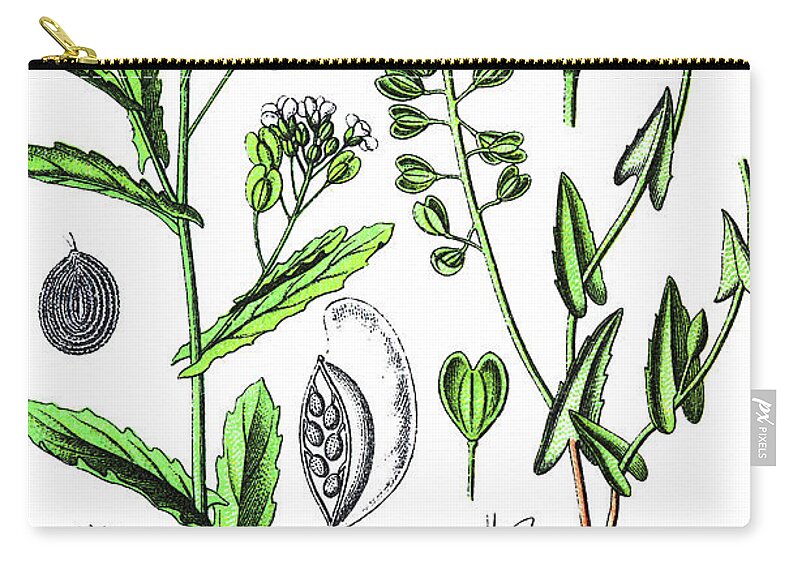The image depicts a change purse or small storage bag set against a completely white background. This realistic photograph has isolated the item, showcasing it with meticulous detail. The purse itself is made of a white fabric, possibly canvas or very soft plastic, and features a black and gold zipper running along the top. The zipper, sewn in with black stitching, has gold brass-colored teeth and a matching slider mechanism. The white fabric is adorned with intricate illustrations of various plants, resembling old lithographs. These black-outlined illustrations are filled in with shades of green, depicting leaves, stem structures, small flowers, and seed pods, including a cross-section of a flower bulb. Additionally, there are both colored and black-and-white drawings of plant elements, highlighting the botanical theme. A small gray text box on the bottom right corner of the purse displays the brand name "PX Pixels" in a neat script logo. This well-crafted and meticulously detailed item appears to be part of an advertisement, likely for online retail, emphasizing its blend of functional design and aesthetically pleasing botanical illustrations.